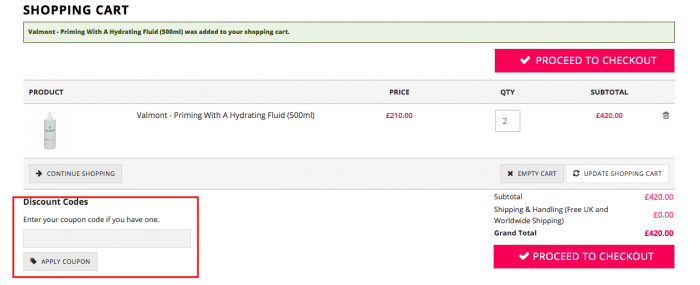A shopping cart displaying a summary of selected items, including two water bottles priced at $428. The subtotal before discounts is shown as $420, with an option to enter a coupon code highlighted in a red box. Shipping and handling are free, maintaining the grand total at $420. The page features two red "Proceed to Checkout" buttons, one at the top right and another at the bottom.